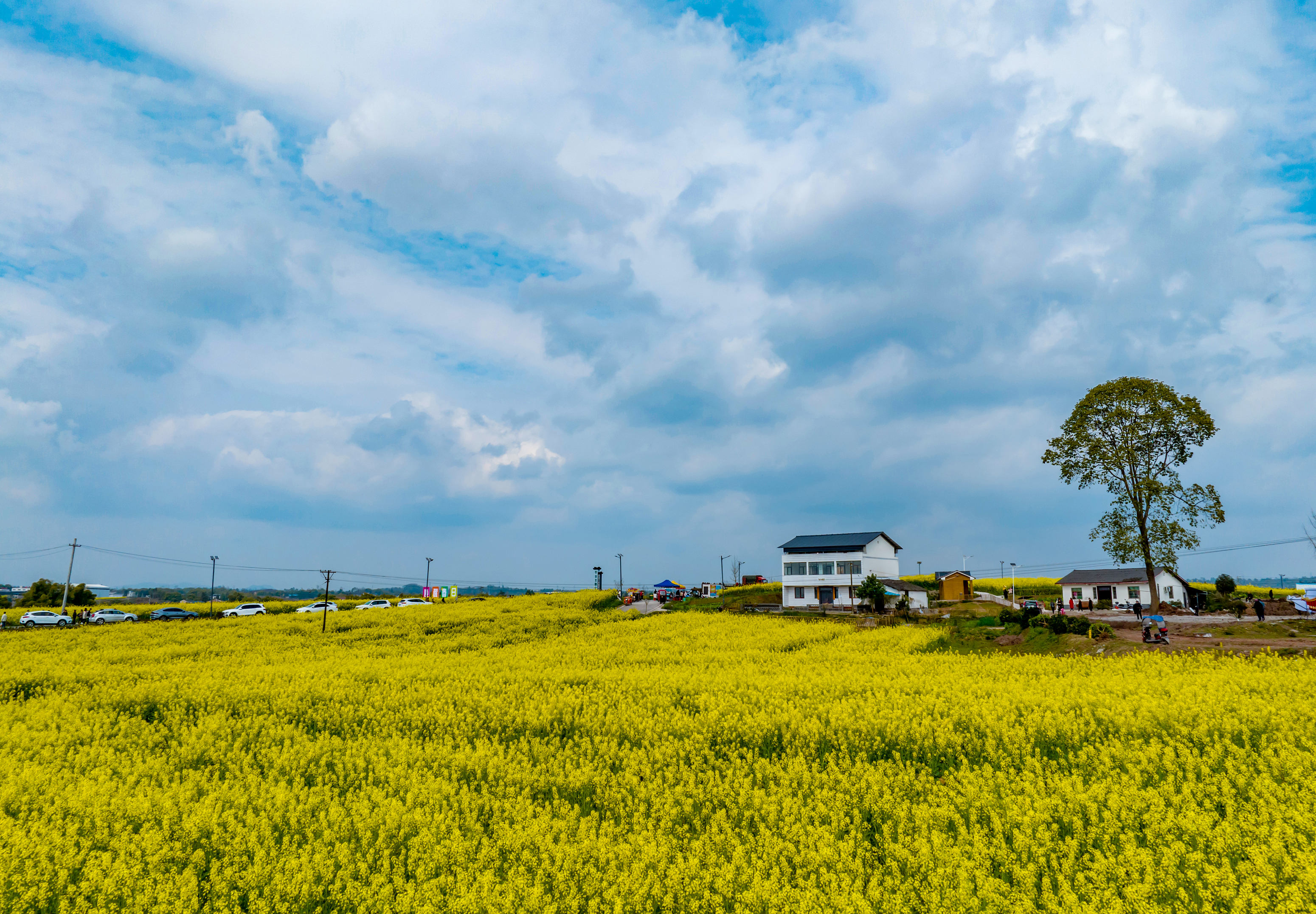The image showcases a breathtaking, wide-angle view of a vast field brimming with mustard-yellow, canola flowers that stretch towards the horizon. Dominating the scene is a strikingly blue sky adorned with highly detailed, bulbous clouds that create a vivid contrast against the vibrant yellow field. On the left side, you'll glimpse a green tree line in the distance, interspersed with telephone poles and wires running along a road. This road features several vehicles, primarily white cars along with a solitary blue one, traveling from left to right.

In the background, there are two main structures: a prominent, two-story white farmhouse with a black roof, and a smaller, white barn situated to its right. On the far right, near another white house with a black roof, a large, sparsely-leafed tree stands tall, partially shading a group of people who appear to be engaged in a playful gathering. The scene is further enriched by patches of green space around the buildings, adding complexity to the heartwarming rural landscape.